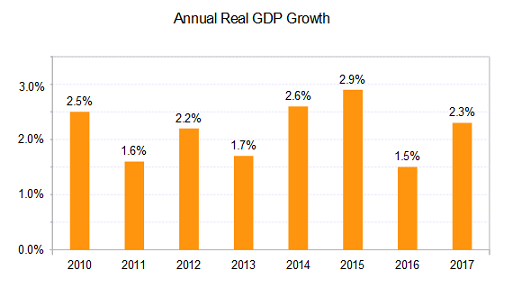This image displays a rectangular bar graph titled "Annual Real GDP Growth" in black text at the top center. The Y-axis on the left indicates percentages with markers at 0%, 1%, 2%, and 3%. The X-axis along the bottom charts the years from 2010 to 2017. Each year is represented by an orange bar indicating the percentage growth: 2.5% for 2010, 1.6% for 2011, 2.2% for 2012, 1.7% for 2013, 2.6% for 2014, 2.9% for 2015, 1.5% for 2016, and 2.3% for 2017. The graph is simple and clean, with no additional elements other than the labeled bars.